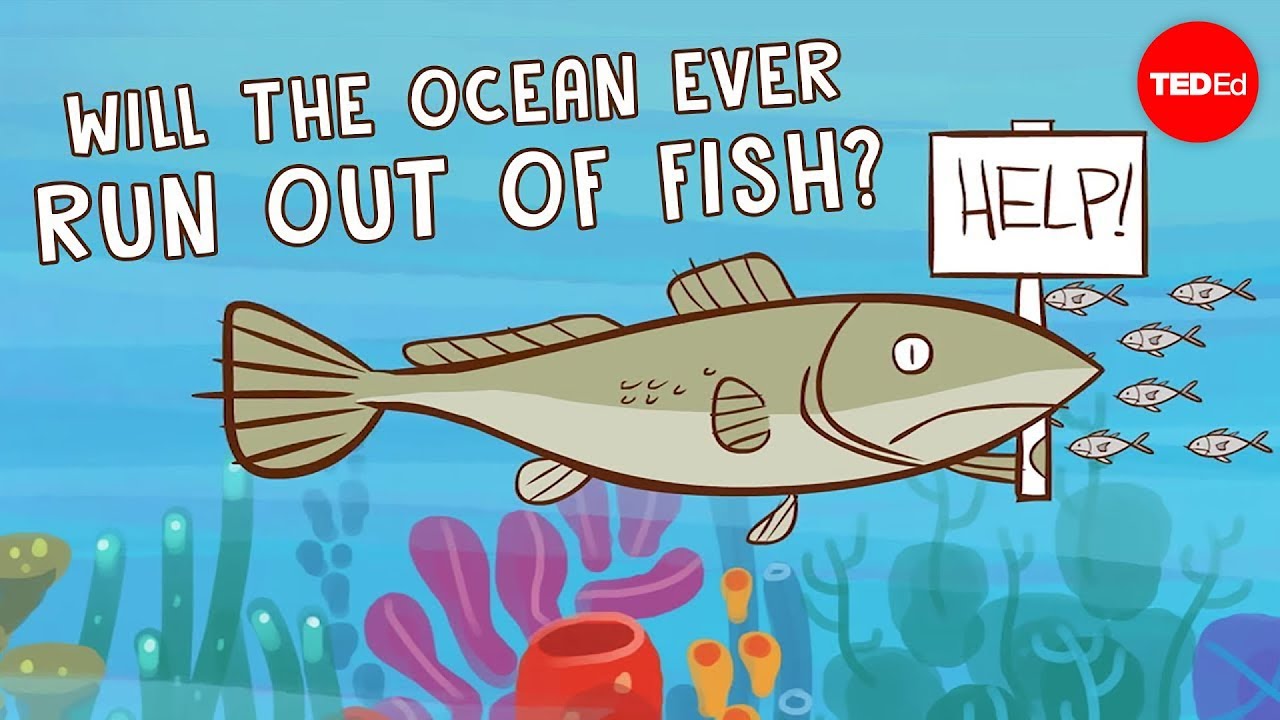In this cartoon-style image, we see a detailed underwater scene featuring a green fish swimming towards the right side, carrying a white sign that reads "Help!" in black text. The fish has a frown on its face, adding to the sense of urgency conveyed by the sign. Surrounding the main fish, there are six other fish swimming in the distance, contributing to the lively marine environment. The ocean water is a vivid blue, and the seabed is populated with various colorful corals and aquatic plants, including green, purple, red, and magenta hues. 

In the upper left corner of the image, white text asks the provocative question: "Will the ocean ever run out of fish?" suggesting a theme of environmental concern. On the upper right corner, a red circle contains the white text "TED-Ed," indicating that this could be a promotional or illustrative image related to a TED-Ed video that explores thought-provoking and educational topics.